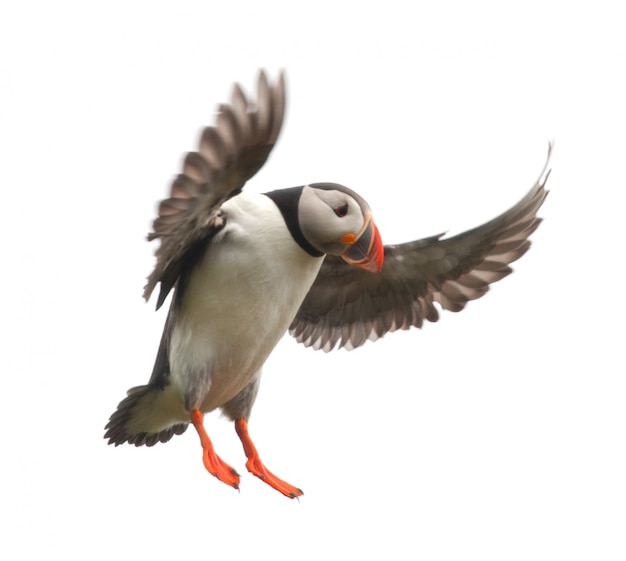This image, set against a white background, features a puffin in mid-flight. The puffin is flying with its wings fully outstretched, showcasing its distinctive coloration and features. The bird's underbelly, chest, and sides are white, contrasting with the black band around its throat and the dark gray to black feathers on its back, head, and top of its tail. The wings are dark gray, with the feathers appearing lighter at the tips. Its beak is strikingly colorful, featuring a mix of bright neon orange, darker orange, light orange, and gray, with white lines marking the transitions between these colors. At the base of the beak is a noticeable yellow spot. The puffin's eyes are dark, surrounded by light gray feathers, and it has an oval-shaped patch of white around each eye. The legs and webbed feet of the bird are an orange to orangey-red hue, and they are positioned as if the puffin is preparing for a landing. The puffin's body appears curved, accentuating the sense of motion and descent.